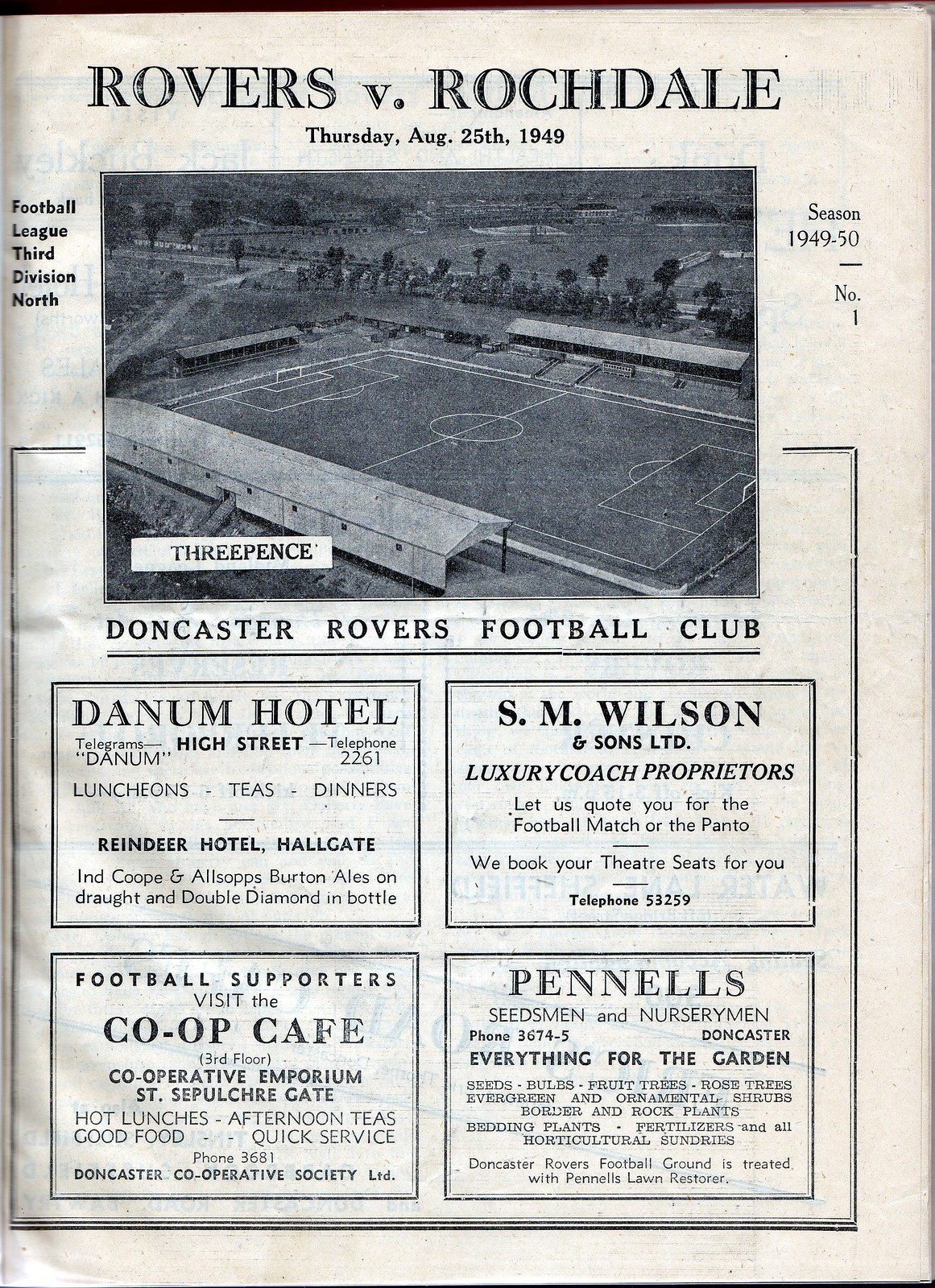The image depicts the cover page of a vintage Doncaster Rovers Football Club program from a match against Rochdale on Thursday, August 25th, 1949. This black-and-white document pertains to the Football League 3rd Division North for the 1949-1950 season and was priced at three pence. Prominently displayed at the top are the team names "Rovers vs. Rochdale," along with the date. The center features an aerial view of the playing field, lined by spectator stands. Below the picture, the name "Doncaster Rovers Football Club" is clearly marked. The lower portion of the page is filled with advertisements: Danum Hotel on High Street offering luncheons, teas, and dinners; Reindeer Hotel on Hall Gate; S.M. Wilson & Sons, Ltd, promoting luxury coach services; the Co-operative Emporium inviting football supporters to its Co-op Cafe on the third floor at Sepulchre Gate; and Pennell's, identified as seedsmen and nurserymen, supplying everything for gardening.